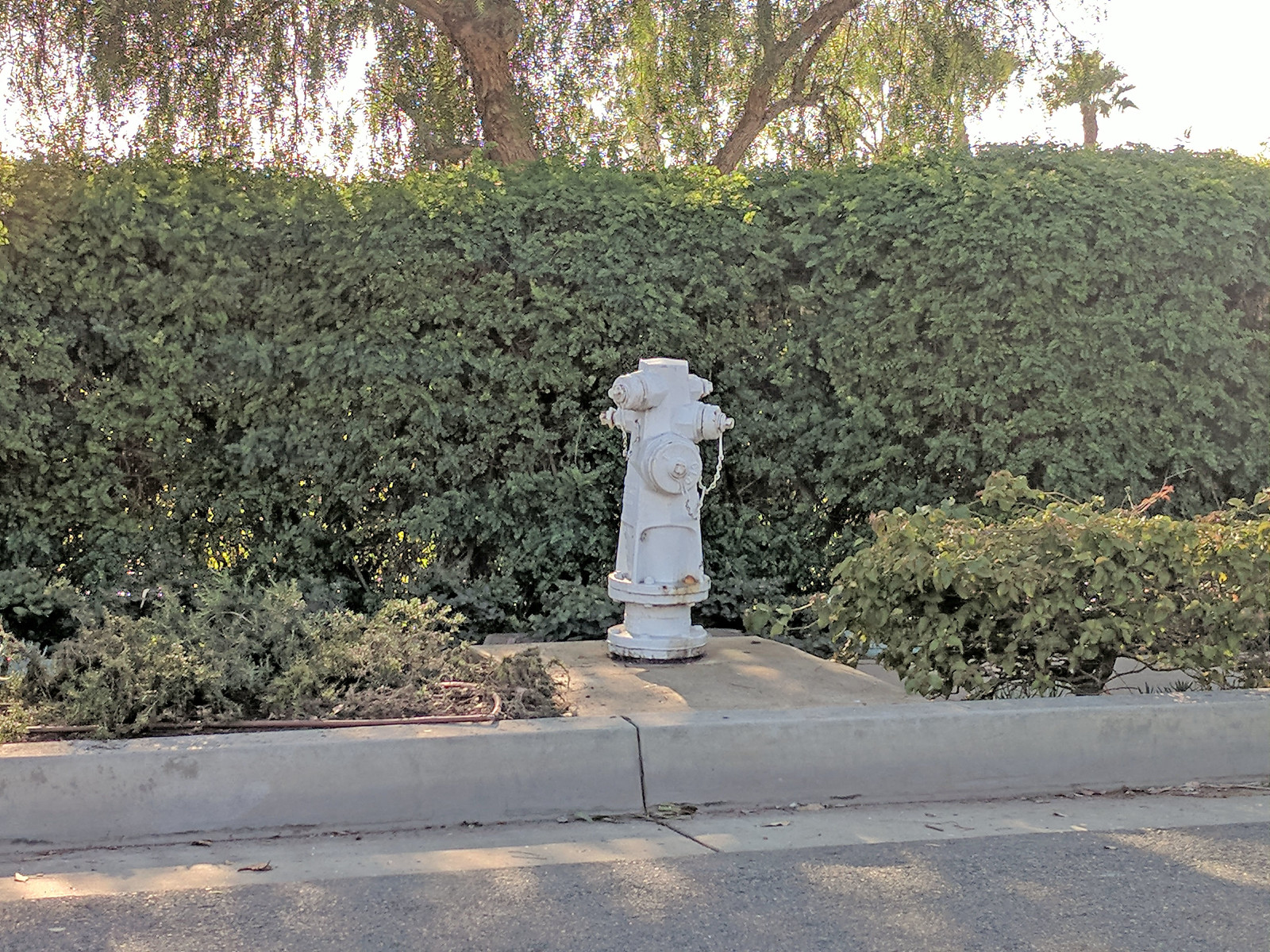In this detailed image description, at the forefront, there's a portion of a road with a tall gray curb. Atop the curb is a gray concrete platform on which stands an old, white fire hydrant bearing various valves, one of which has a chain attached to it. Flanking the fire hydrant on both left and right sides are small patches of green plants. Behind the hydrant extends a tall, well-maintained green hedge that occupies the entire background from left to right, showcasing a consistent height and uniform appearance. This hedge features predominantly dark green leaves interspersed with lighter green areas and a few yellow spots. Above the hedge, mature trees with thick trunks rise, their green foliage creating an overhang. Beyond the trees, a clear white sky is visible, completing the serene and lush backdrop of the scene. The ground in front of the curb has some white markings, adding subtle detail to the image.